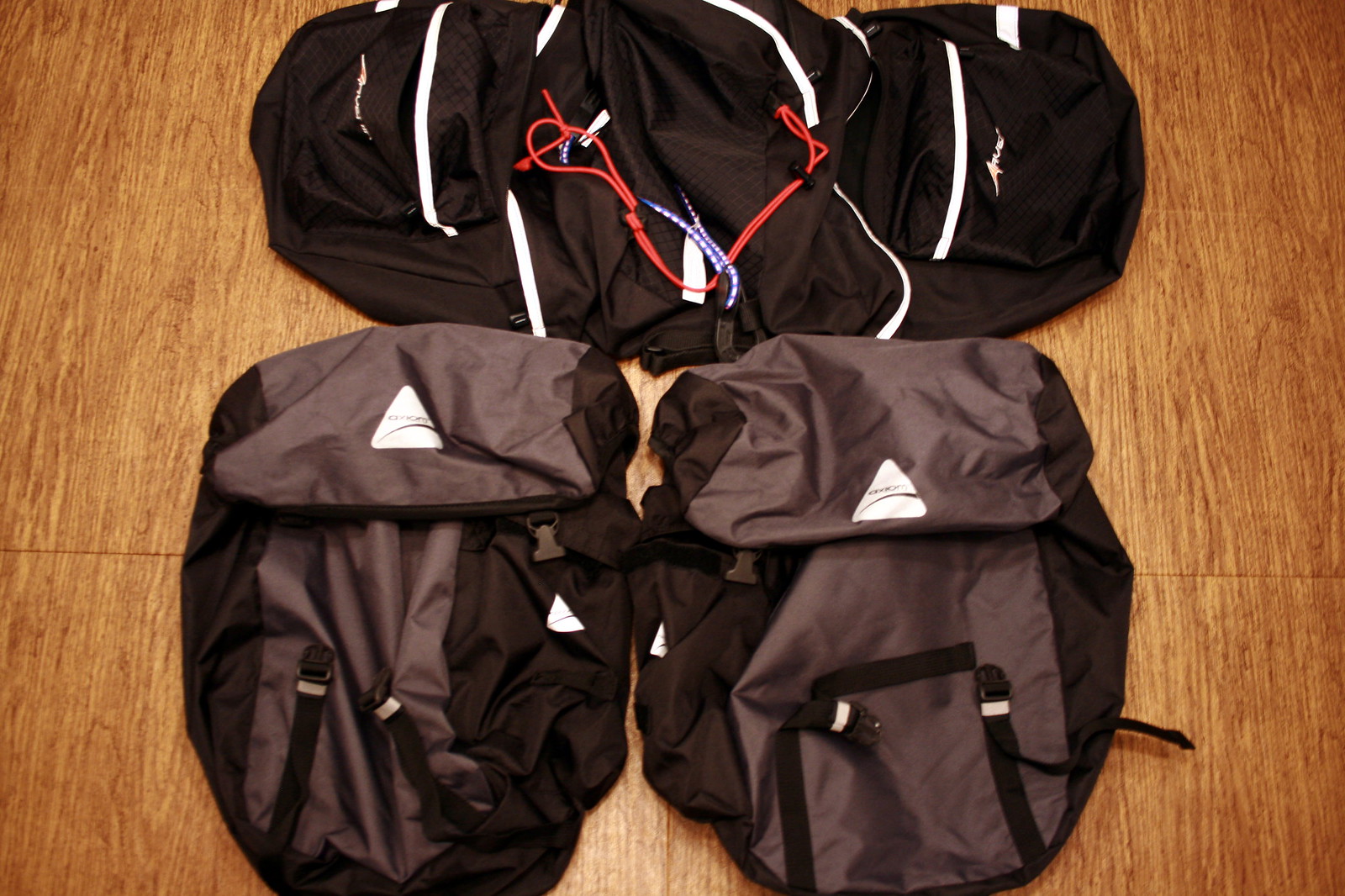The image captures a neatly arranged set of four backpacks on a light brown wooden floor. The two backpacks at the bottom are identical, featuring a design with dark gray centers flanked by black sides, and multiple belt buckles with the ends at the bottom and clasp parts higher up. Each bottom backpack has a small white triangle with an unreadable logo on the top flap. The two top backpacks are black with small white stripes extending along the sides and a prominent red cable draped over them. These upper backpacks also have a blue and white rope interspersed with the red cable. All the bags are slightly deflated and have visible crinkles, enhancing their detailed texture in the photograph. The wood floor, with its visible seams and grain, adds a warm background to the scene.